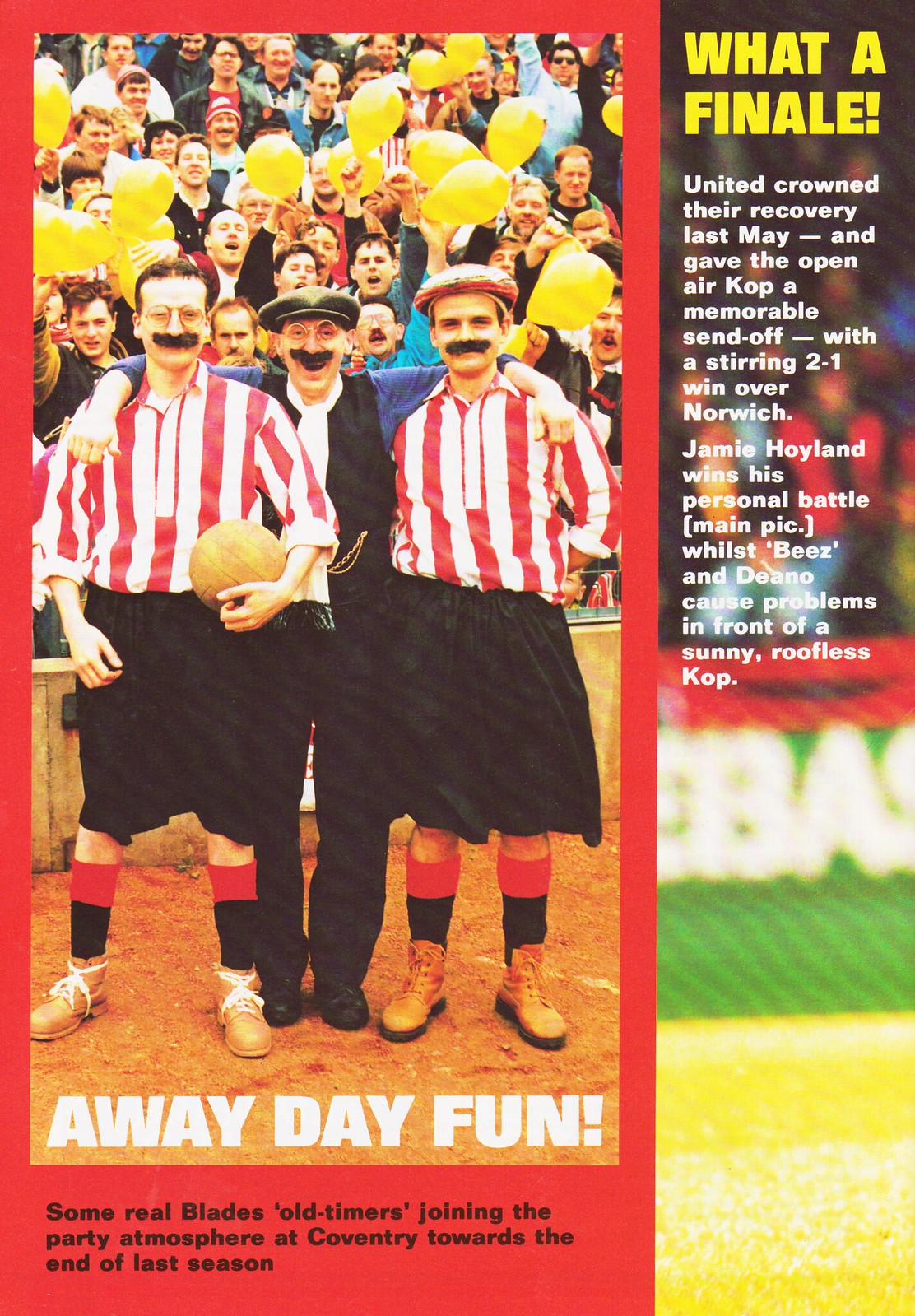The image captures a vibrant scene from a magazine page featuring a lively crowd and three central figures amid a celebratory moment. The background is bright with a mix of yellow and green hues, though it's slightly blurry and hard to fully discern. Dominating the right side is a vertical rectangular box with bold text. At the top, in yellow capital letters, it reads "WHAT A FINALE." Below, white text narrates, "United crowned their recovery last May and gave the open-air Kop a memorable send-off with a stirring 2-1 win over Norwich. Jamie Hoyland wins his personal battle (main pick), whilst Bees and Dino cause problems in front of a sunny, roofless Kop." 

To the left, a zoomed-in photo showcases three men, each sporting a jovial fake mustache. The central figure, flanked by the other two, wears a black and blue suit with a white necktie and a vest. He has his arms around the shoulders of the other two, who are garbed in red and white vertically striped shirts and black pants, resembling referees. The left referee holds a ball in his hand. All three appear joyous, with the main man smiling broadly, highlighting his large black mustache.

In the background, a crowd exudes excitement, some waving or wearing yellow hats and holding up yellow balloons, creating an atmosphere of celebration. The bottom caption reads, "Away day fun: Some real blades, old timers, joining the party atmosphere at Coventry towards the end of last season."